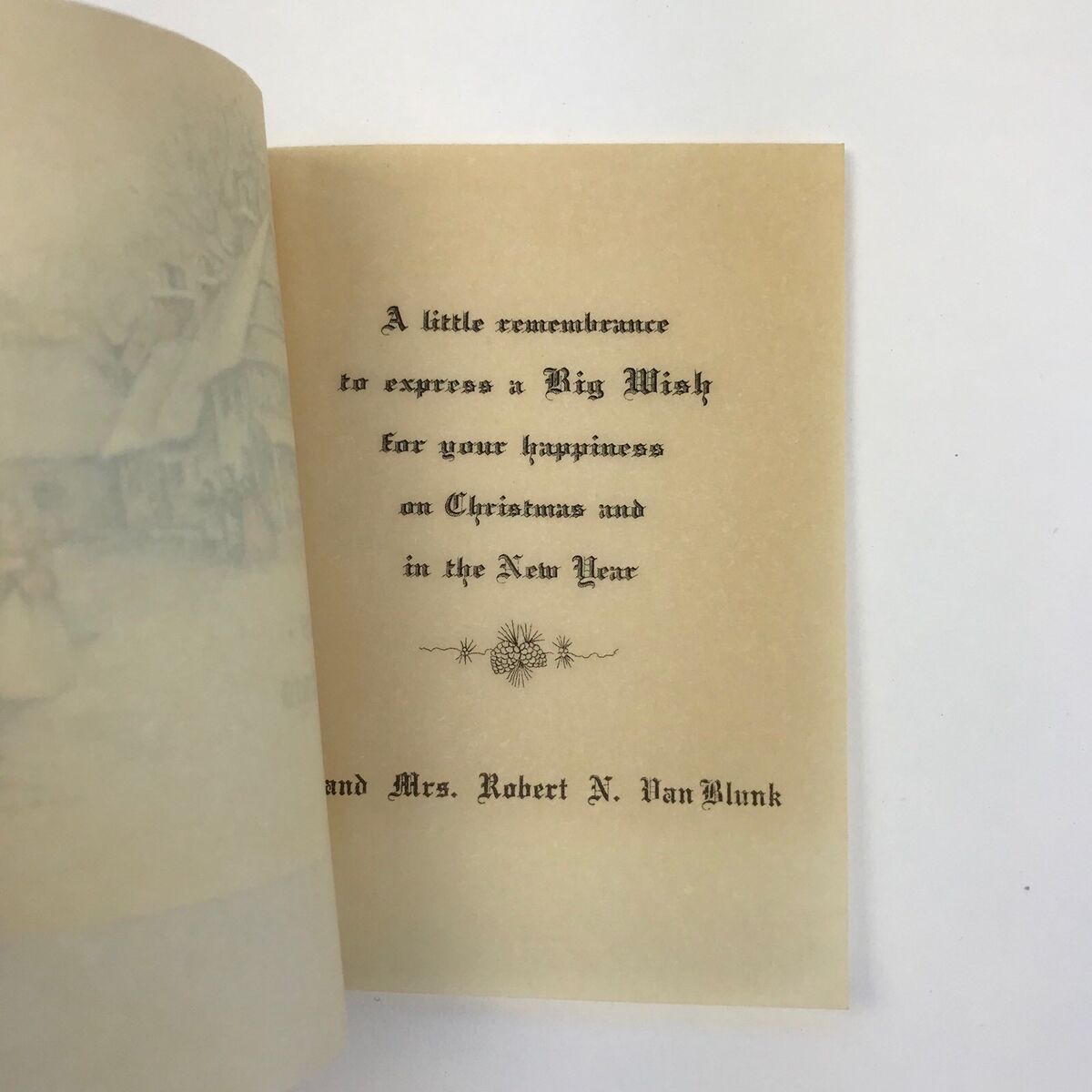This image features an aged, ivory-colored Christmas card that appears to be crafted on parchment-like paper. The card is open, revealing an elegantly written message in a bold, black Old English type font. The central text reads, "A little remembrance to express a big wish for your happiness on Christmas and in the new year." Below this message, there is a delicate design that resembles small pine cones surrounded by stars. At the bottom of the text, the card is signed, "Mr. and Mrs. Robert N. Van Blunk."

Peeking through the partially opened front cover of the card, there is a subtle depiction of a serene winter scene featuring houses and trees blanketed in snow. The card rests on a white surface, and a tiny black speck is noticeable in the bottom right corner of the image.